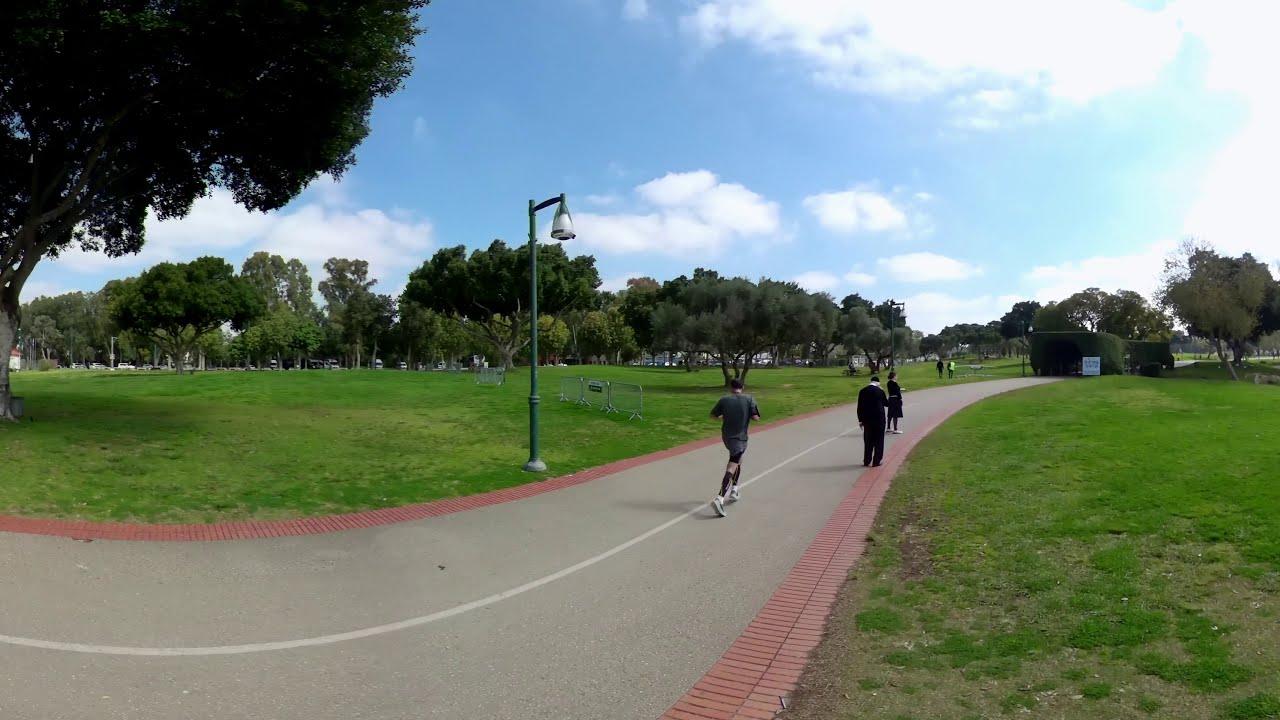The image depicts a vibrant park scene under a blue sky adorned with white, fluffy clouds. A gray, bricked walking and jogging path with a white center line snakes from the bottom left to the center right of the image. The path is bordered by red bricks on both sides and is flanked by expansive green grass fields and tall, lush trees lining the perimeter. A lamppost stands on the left side of the path, casting light over the area.

In the foreground, a man is captured mid-jog, dressed in a blue shirt, gray shorts, knee-high black socks, and trainers. Close behind him, two people are walking and appear to be engrossed in their phones, both clad in black clothing. Further ahead, an elderly man in all black and a woman walk leisurely along the path. Additionally, two more figures can be seen in the distance, strolling through the grassy areas of the park.

The overall setting is lively with abundant greenery and a well-maintained pathway that offers different activities for joggers and walkers alike. There is some signage in the distance, though its details are not discernible. This peaceful daytime scene is enhanced by the presence of numerous trees and ample natural beauty.